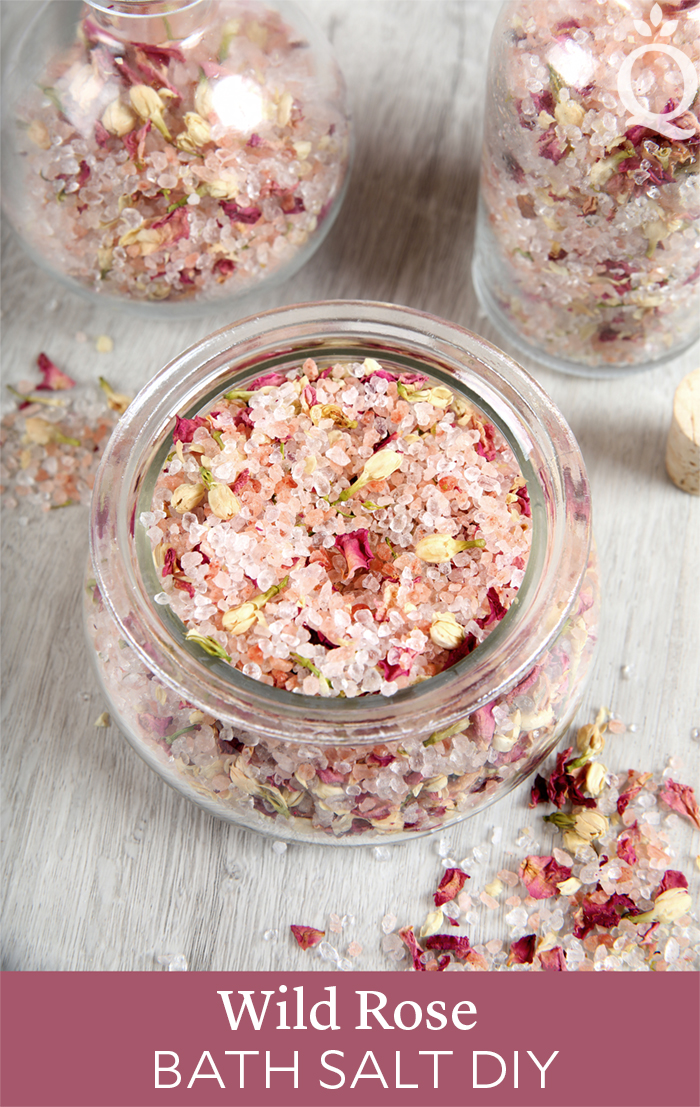The image is a vertically rectangular, full-color photograph taken indoors during the day, utilizing both natural and artificial light. At the very bottom of the image, there is a burgundy-colored border featuring white text that reads "WILD ROSE BATH SALT DIY." This banner sits on top of a white, painted wooden tabletop that appears grainy in texture. The focus of the photograph is three glass jars filled with multicolored bath salts, prominently featuring red, pink, yellow, and strawberry-like crystals. These jars are neatly arranged above some loose sprinkles of the same salts scattered on the surface. In the bottom right corner, there’s a small pile of these colorful crystals, adding to the decorative appeal. Additionally, the upper right-hand corner of the image is marked with a watermark—a pink letter "Q" placed over one of the jars.